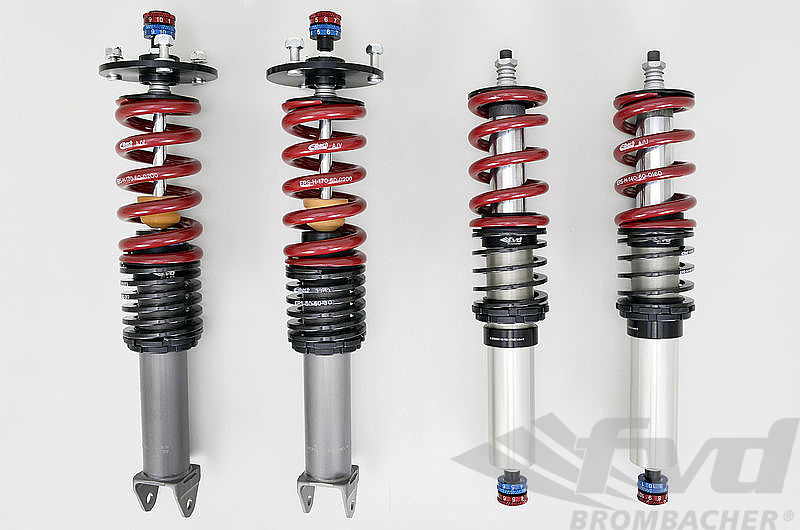The photograph features four Eibach shock absorbers positioned vertically against a light gray background, each meticulously detailed and well-lit. On the left, two larger shock absorbers are showcased, each comprising black coils tightly wound near the base and more widely spaced red coils above them. A thin, silver cylindrical tube stretches from a lower U-shaped attachment bracket through the black coils to the top, where it finishes in a round black plate secured with bolts. A key highlight in the bottom area is the dual round circles—one red, beneath and an upper blue—that resemble components for further assembly.

On the right, two shorter shock absorbers are similarly organized but are comparably narrower. These also feature tightly wound black coils in the middle and more spacious red coils above. However, they differ at the base with a distinct red and blue capped-end instead of the U-shaped bracket, suggesting different functionalities or attachment methods. The top ends mirror the left pair with cylindrical tubes and threaded nubs.

In the lower right corner of the image, the logo "FVD" is positioned above the bold text "BROMBACHER," enhancing the mechanical, professional appeal of the photograph.